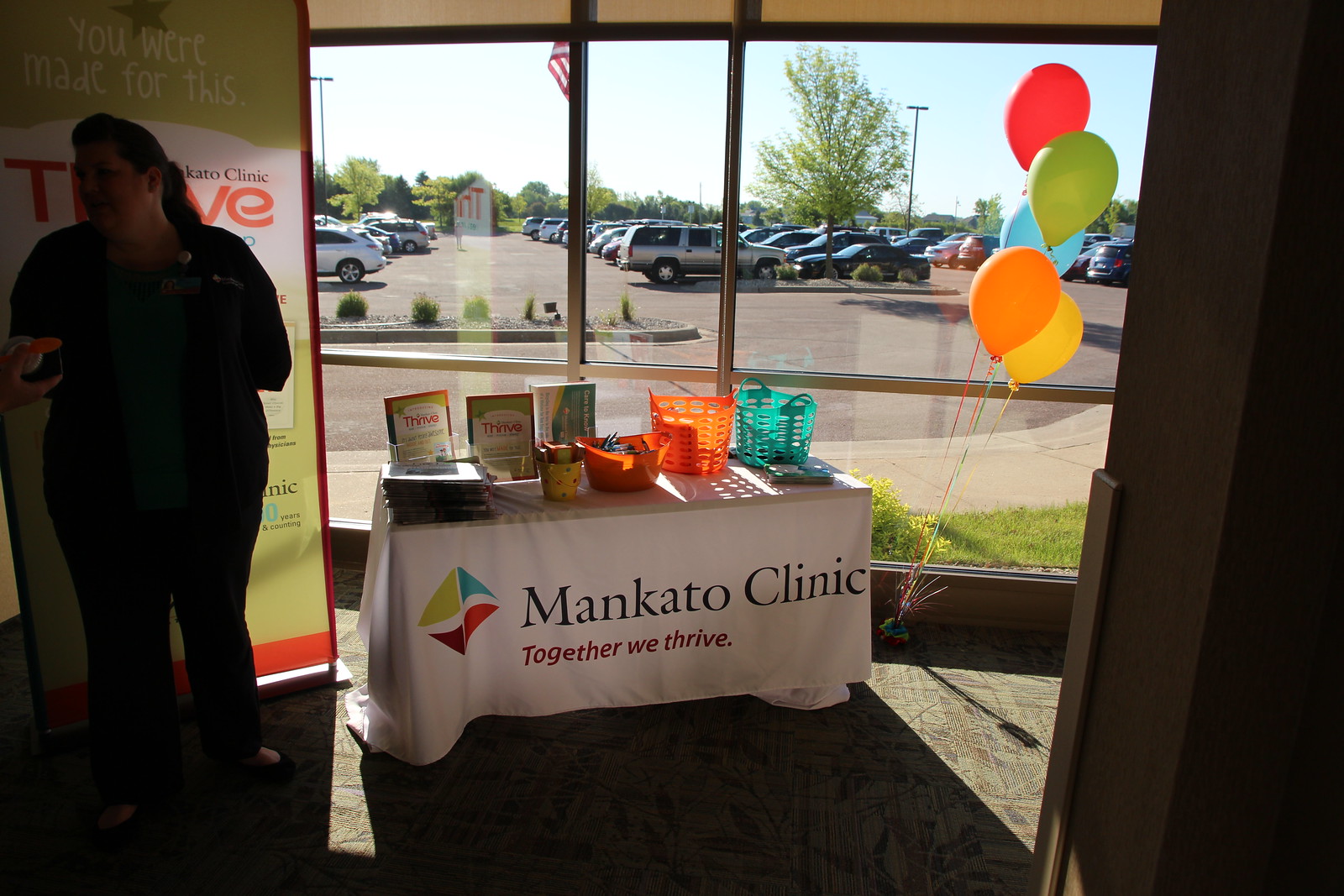The photograph captures a detailed scene inside a building, likely at a trade fair or job fair. Centered in the image is a small rectangular table draped with a white tablecloth. The tablecloth displays a colorful logo on the left front, consisting of diamond-shaped segments in lime green, turquoise, magenta, and red. Large black text next to the logo reads "Mankato Clinic," with smaller pink text underneath stating "Together We Thrive." Atop the table, there are several multicolored books and baskets in orange and teal, arranged towards the right. To the right of the table, a cluster of balloons in red, green, orange, and yellow is tethered to the floor.

Behind the table is a large glass window, offering a view of a gray-paved parking lot bustling with cars. Beyond the lot is a road, some grass, a gray sidewalk, and a few trees with bright green leaves under a light blue sky. The left side of the image features a person standing in shadow, making details difficult to discern; however, they appear to be wearing dark scrubs and have long, dark hair with arms behind their back. A large green, white, and orange sign is positioned near this individual.

The overall ambiance of the image suggests a busy, daylight setting, with various promotional items and decorations hinting at a welcoming and organized environment.